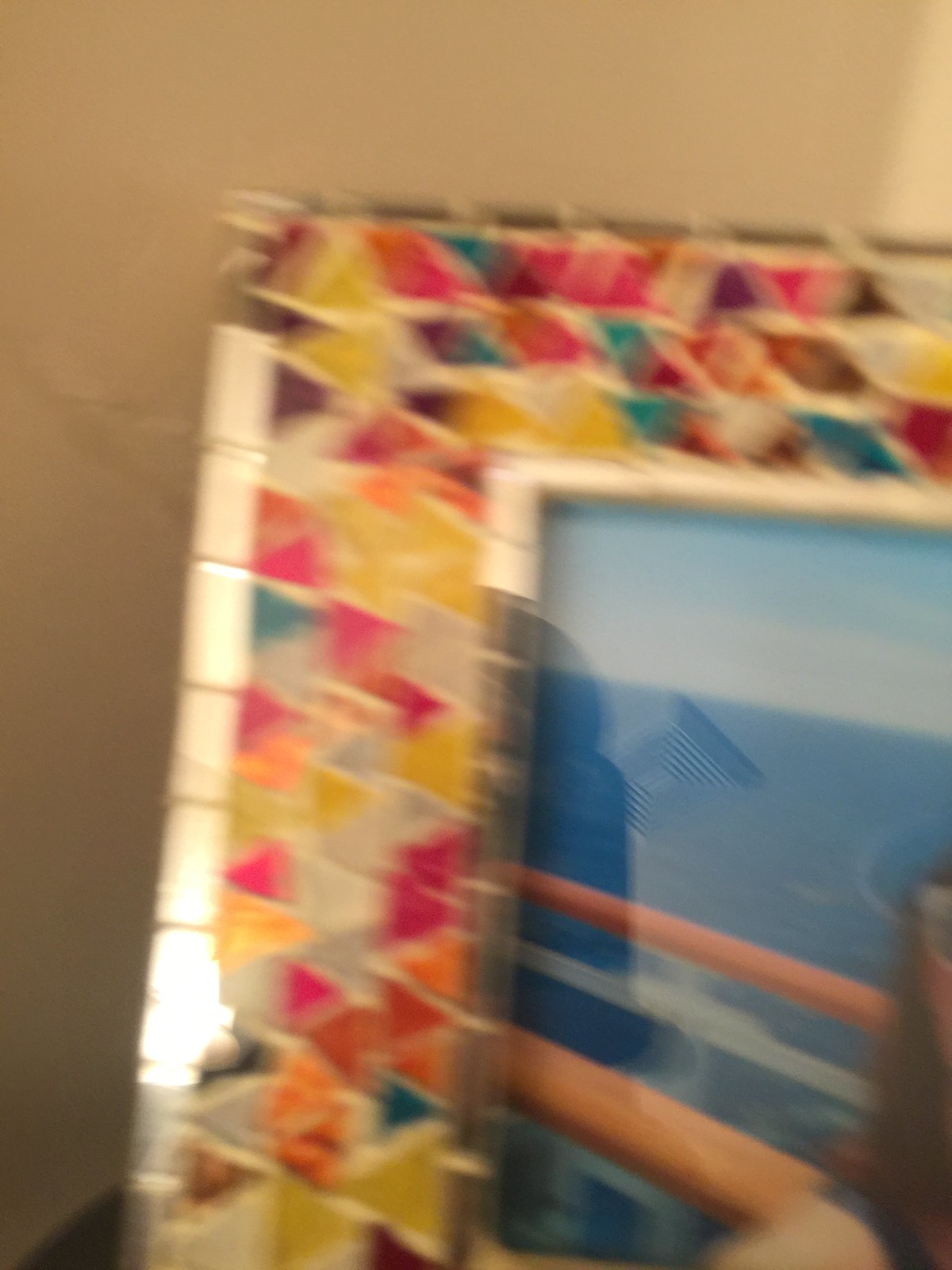This image features a unique and vibrant piece of artwork, characterized by an assortment of elongated, kite-shaped, and triangular tiles meticulously layered in a colorful collage. The geometrically varied elements are composed of vivid hues, applied in segments and sections, forming a dazzling mosaic pattern. These tiles, resembling chiclet-like edges, collectively create an elaborate, out-of-focus frame that adds an abstract yet compelling quality to the image.

In the frame's center, there is an intriguing, though blurry, photograph that appears to capture a serene maritime scene. The photo seemingly depicts a view looking out at the sea, framed by the orange and cream-colored railings of what could be a cruise ship. The hazy horizon lines blend softly with the green sea, invoking a sense of peaceful vastness. The entire composition rests against a tan background, giving the impression of a colorful frame perched on a shelf, holding a distant and dreamy seascape. The overall out-of-focus nature of the image invites viewers to engage their imagination, squinting to discern the beauty and tranquility that the photo portrays.